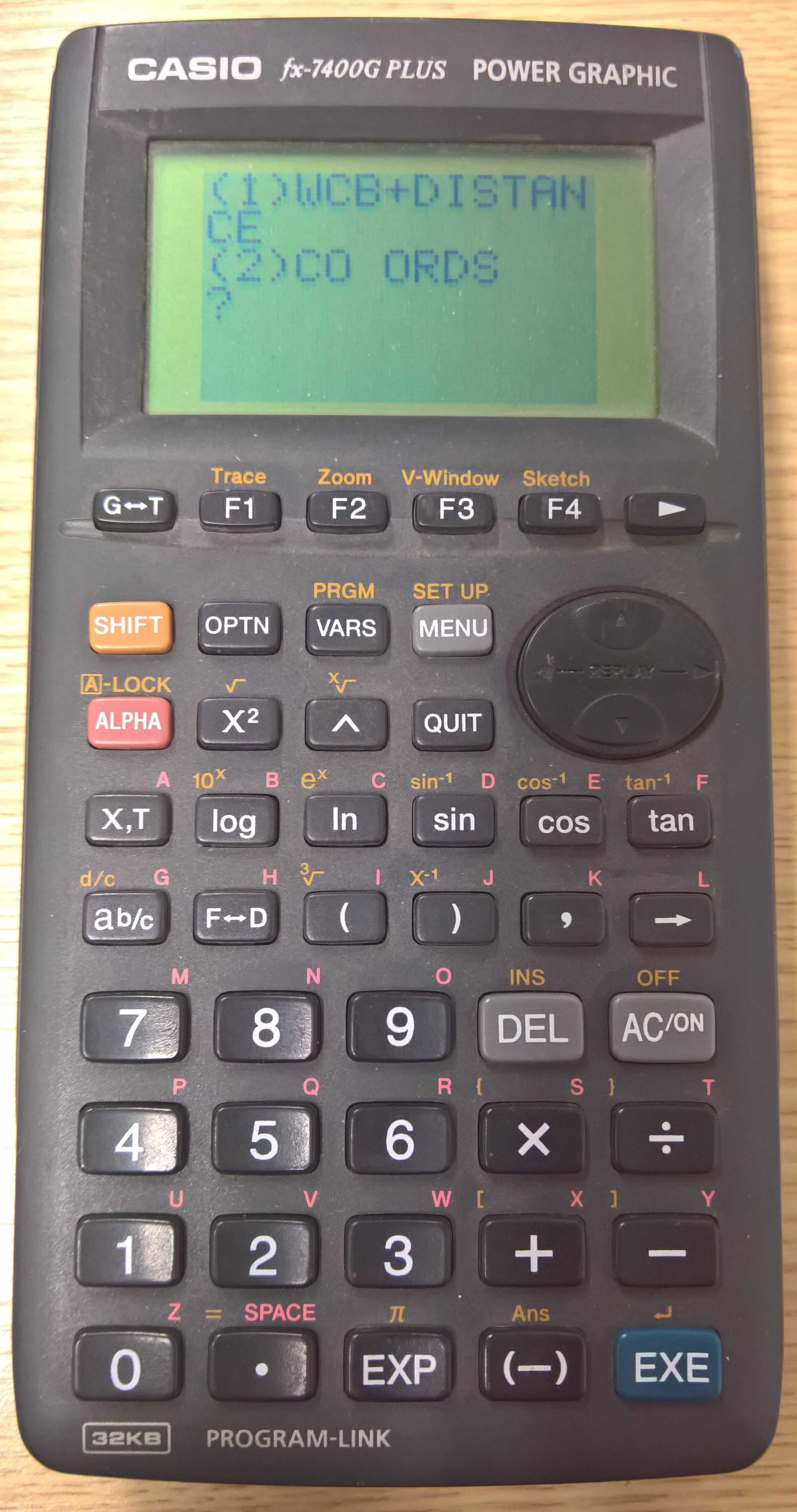The image showcases a Casio FX-7400G Plus Power Graphic graphing calculator, which takes up the entire frame against a brown table or counter background. The calculator is black with numerous black buttons labeled in white, with several special function buttons highlighted in colors: the Shift key in orange, the Alpha key in pink, and the EXE button in dark teal blue. At the top of the device, "Power Graphic" is prominently displayed in gray font. The calculator's screen displays the text: "(1) WCB + DISTANCE (2) COORDS". Among the various keys, categories like Trace, Zoom, V-Window sketch, Shift, Option, Variables, and Menu can be found, as well as standard mathematical function keys such as those for logarithmic, sine, cosine, tangent, and square root operations. Underneath all the buttons, a small rectangle contains the text "32 KB Program-Link".